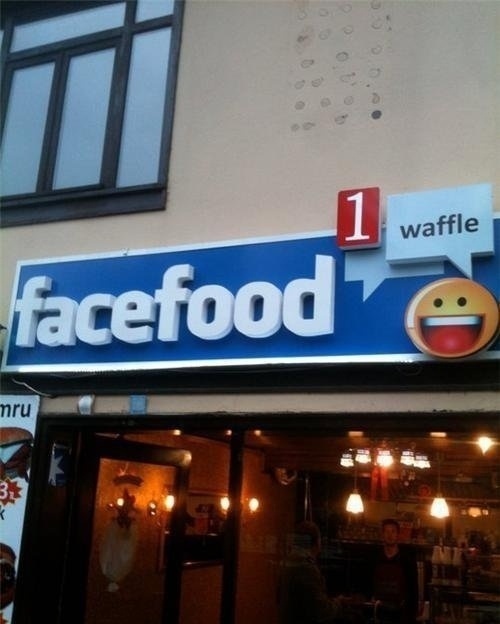The photograph captures the front of a restaurant situated in the bottom half of a tan-colored building. The top left corner of the building showcases a multi-pane window with a black frame. The restaurant's facade features a large glass front and an open glass door, also framed in black, allowing a glimpse inside where some suspended lighting fixtures can be seen. Prominently displayed above the storefront is a blue rectangular signboard with a white border. The signboard boldly reads "FaceFood" in white, large race text, clearly a playful nod to the social media platform Facebook. To the right of the text on the signboard, a cheerful smiley face is depicted alongside a blue square speech bubble that reads "waffle" in black text, suggesting the restaurant specializes in waffles. The image includes a variety of colors such as tan, gray, blue, white, yellow, orange, red, and black, adding vibrancy to the scene. Additionally, part of a cut-off menu can be seen on the left side of the glass front. The setting is outdoors, looking into a bright and inviting restaurant with customers inside.